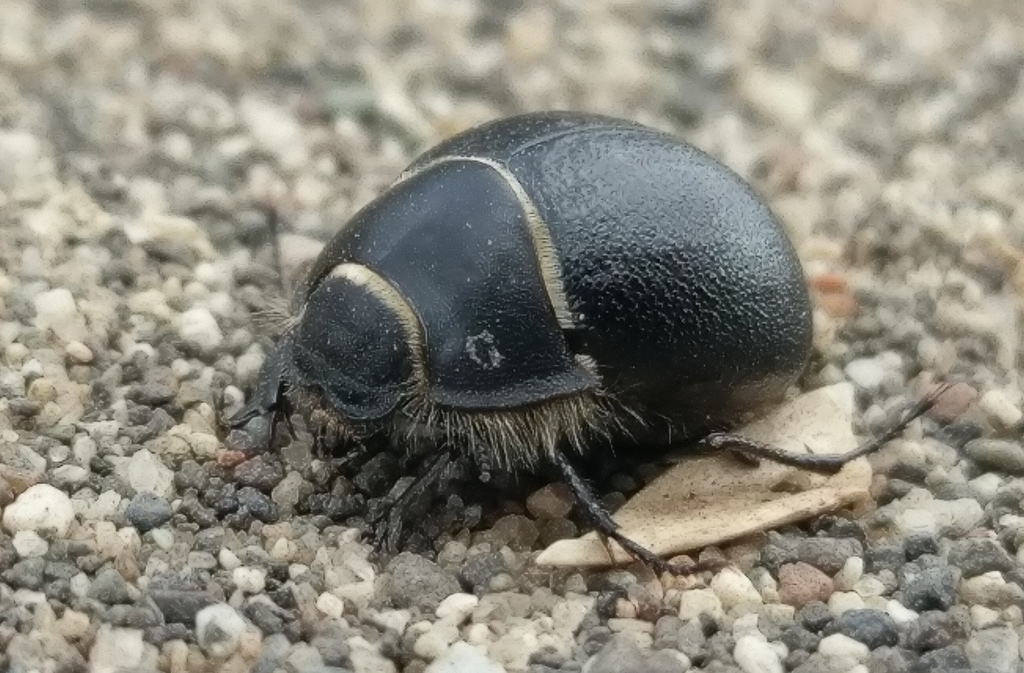The image is a close-up photograph of a small beetle with a distinct, hard shell. The beetle's body is primarily black, with a shiny, curved carapace that features a line of yellowish-tan separating the back from the front. The front part of the beetle's body, housing its head, is a less shiny, flat black, and has a small protrusion resembling a nose. Thin, hair-like projections are visible underneath the front part of the body, along with at least three spindly legs equipped with small hooks or needles for climbing. The beetle is positioned centrally in the image, oriented towards the lower left, with its head on the left side and its exterior back shell on the right. It rests on a bed of gravel-like pebbles of varying colors, including white, gray, and hints of red. To the right of the beetle, amidst the pebbles, there's an irregularly shaped white object that is significantly larger than the surrounding rocks. The background and setting suggest a heavily zoomed-in perspective, highlighting the intricate details of the beetle's shell and the texture of the gravel.